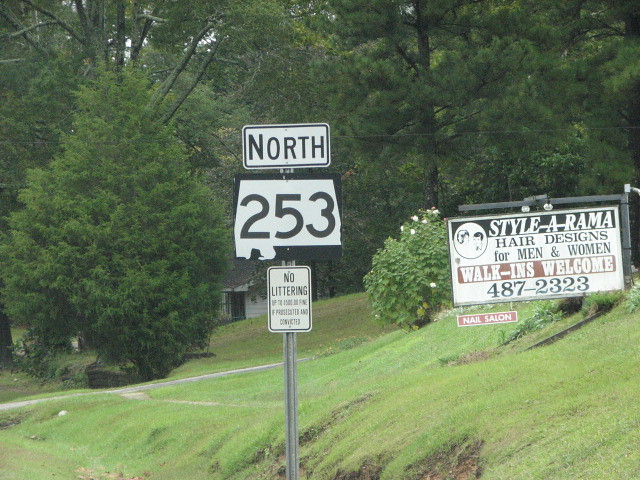A street sign reads "North 253" with a smaller sign beneath it that states "No Littering." Nearby, a small billboard stands by the roadside amidst a grassy, slightly inclined area. The sign advertises "Stylorama Hair Designs for Men and Women" with a note that walk-ins are welcome and also mentions a nail salon. Surrounding the sign, there is an abundance of greenery, including large trees and bushes. The lawns in the area appear somewhat unkempt, and the overall atmosphere is gloomy with overcast skies.